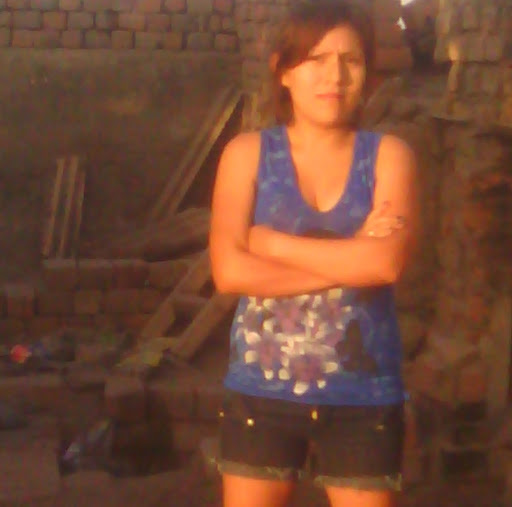This is a blurred image of a young woman, potentially anywhere from a teenager to her early 30s, standing in front of a deteriorating brick wall or possibly an outdoor brick fireplace. She has light skin and brown hair that is tied back. Her expression is a mix of suspicion and scorn, directed towards the camera. She is dressed in a blue sleeveless tank top adorned with a delicate design of flowers and butterflies, and black jean shorts that are rolled up, featuring a few gold buttons. Her arms are crossed over her chest. The background is cluttered with various wooden items leaning against the wall, and some bricks have detached and fallen to the ground, suggesting a state of construction or decay. The image is cropped at mid-calf, making it difficult to determine other details.